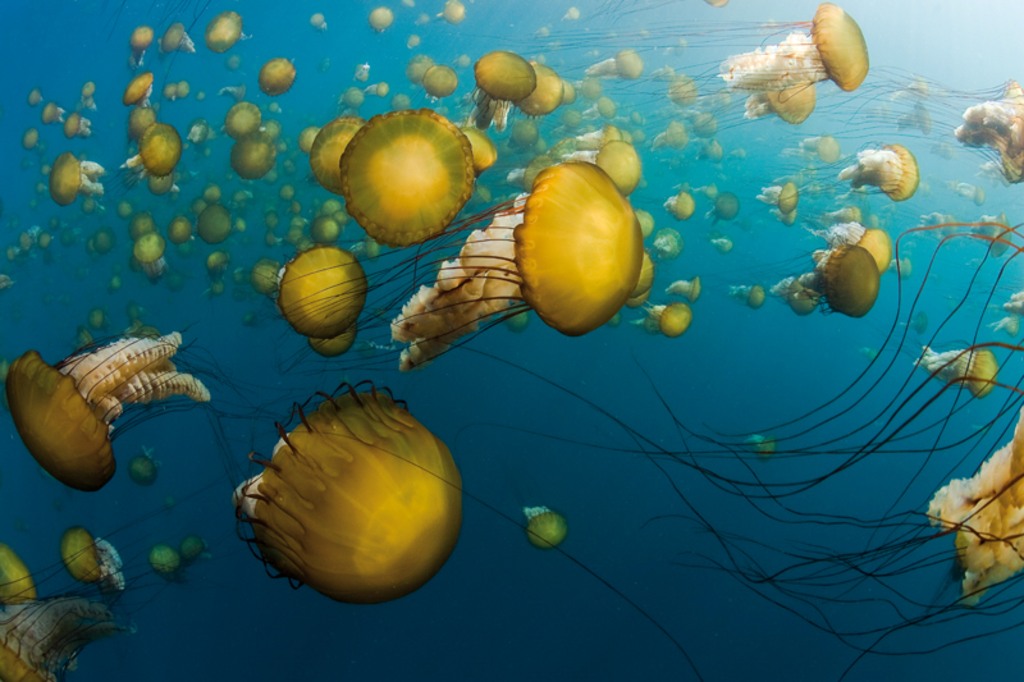The image captures an underwater scene brimming with a school of jellyfish, all of which are glowing in rich orange and yellow hues. These ethereal creatures, numbering likely in the hundreds, are presented in various dynamic forms as they float, predominantly moving to the left while a few appear to swim forward. Each jellyfish boasts a semi-transparent cap and long, dark brown or black tentacles trailing behind, complemented by meaty white strands. The water enveloping them is a slightly murky teal-blue, yet it maintains an almost crystal clarity free of debris. Sunlight illuminates the upper right corner, casting a bright glow across the scene. Despite its photographic elements, the image has an overly smooth texture, suggesting it may be an AI-generated artwork rather than a true photograph.